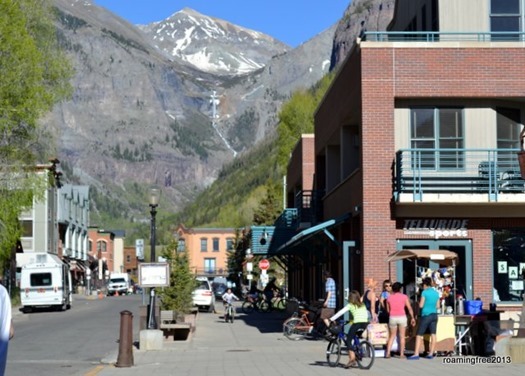This photograph captures a picturesque street scene in a small town nestled against the background of a large gray mountain, topped with scattered white spots and surrounded by a vibrant blue sky. The foreground is bustling with activity, showcasing a combination of urban life and scenic beauty.

On the right side of the image stands a prominent two-story red brick building with the sign "Telluride Sports" above the door, indicating a commercial establishment or possibly a restaurant or bar. The building features blue railings on its second-story balconies and a sidewalk filled with people—some sitting, others standing around a booth, and a girl biking along the walkway. Next to this structure is another brick building with green or light blue railings and an awning, partially cast in shadows where children are seen riding their bikes.

Moving left, there are more buildings, including a notable brown brick building with a few levels and green or light blue railings on its balconies. Vehicles, including white trucks, cars, a bus, and a truck, populate the street, which runs straight towards the mountain. A sign with a black pole and lamp is placed near the road on the left side with some unreadable writing on it. 

Beyond the town, nearer the base of the mountain, are clusters of dark green trees dotting the landscape, and what appears to be a road winding through the middle levels of the hills. The left side of the image also shows additional brown and gray brick buildings, along with parked cars and more greenery, creating a well-balanced composition of structures and natural elements.

In essence, this idyllic snapshot effectively blends the charm of a lively town with the majestic serenity of the mountainous backdrop.